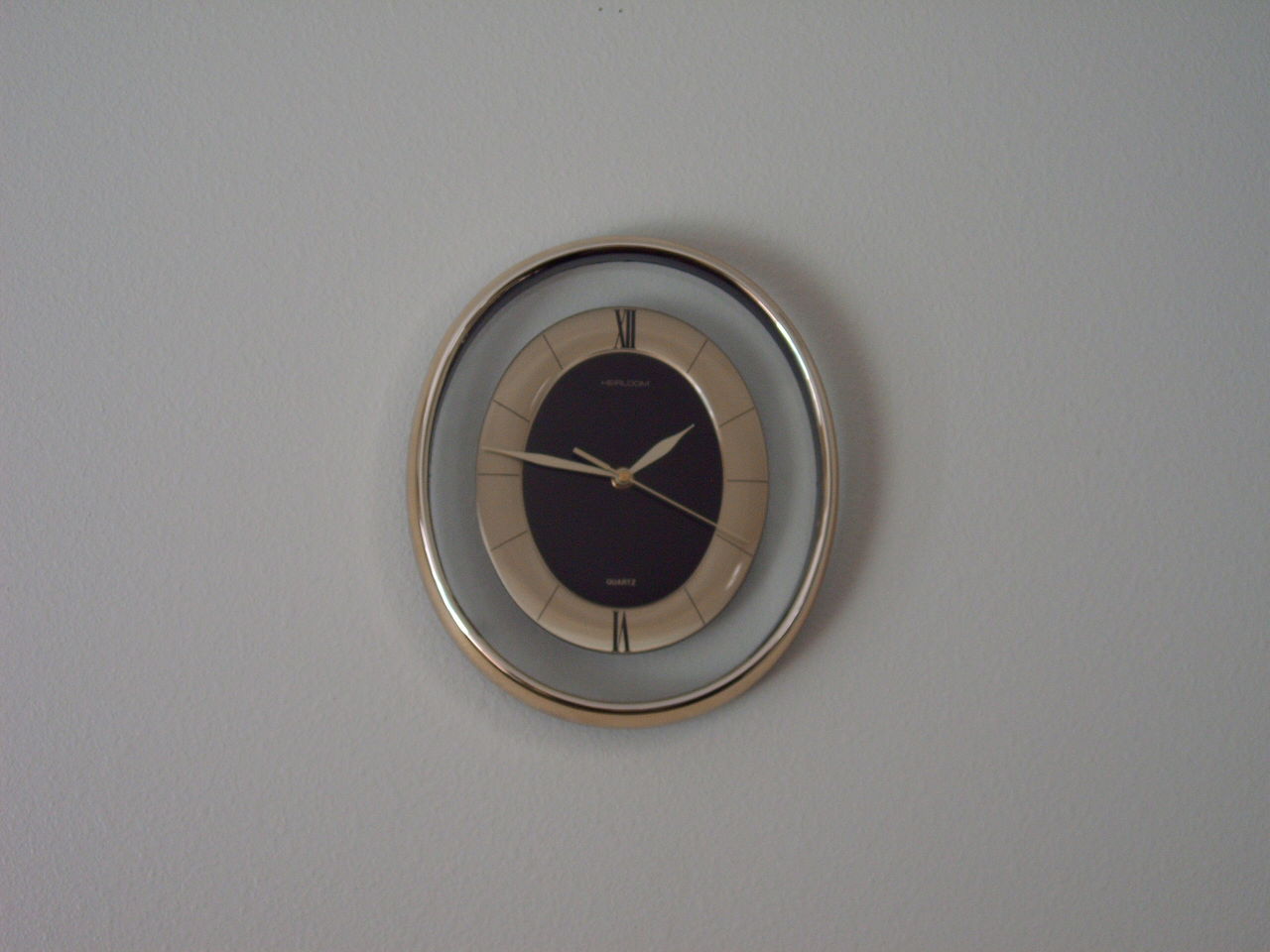The photograph depicts an analog clock mounted on a light gray wall, creating a striking contrast. The clock's design exudes a modern aesthetic with its metallic elements. It features several concentric circles, starting with a thin outer ring made of chrome or brushed nickel, followed by a translucent glass pane through which the wall is visible. Inside the glass is another thicker metallic ring. The clock face itself is black and minimalist, displaying only two Roman numerals at the 12 and 6 o'clock positions, with fine lines marking the other hours. The hands of the clock, including the small hand, large hand, and second hand, are a delicate beige color. The photographed time indicates approximately 1:47. The lighting in the image is relatively dim, suggesting it may have been taken under an overcast sky or in a poorly lit room, softening the overall visual tone.